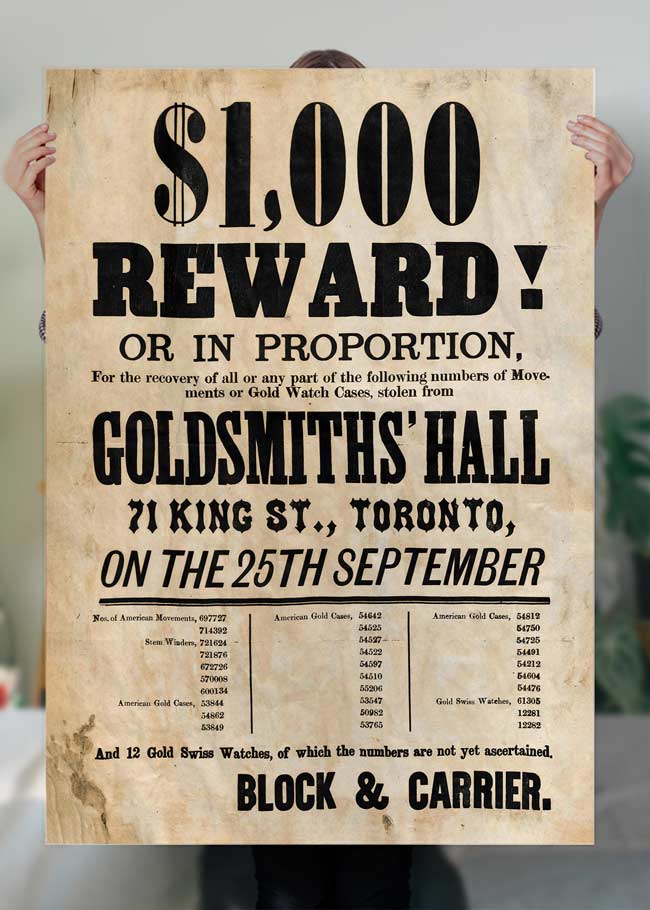A person, mostly hidden behind a large, aged poster, holds it up with only the top of their head and hands visible. The poster, weathered and stained to appear vintage, offers a "$1,000 reward or in proportion for the recovery of all or any part of the following numbers of movements or gold watch cases stolen from Goldsmiths Hall, 71 King Street, Toronto on the 27th of September." The poster features three columns listing different serial numbers and brands of stolen watches, although the text is not entirely legible. Particular emphasis is given to "12 gold Swiss watches of which the numbers are not yet ascertained," followed by a note on "Block and Carrier." The paper exudes an old, dirty gold color, hinting at a historical or gold rush theme, styled as an advertisement promising a reward for the recovery of stolen gold watches.